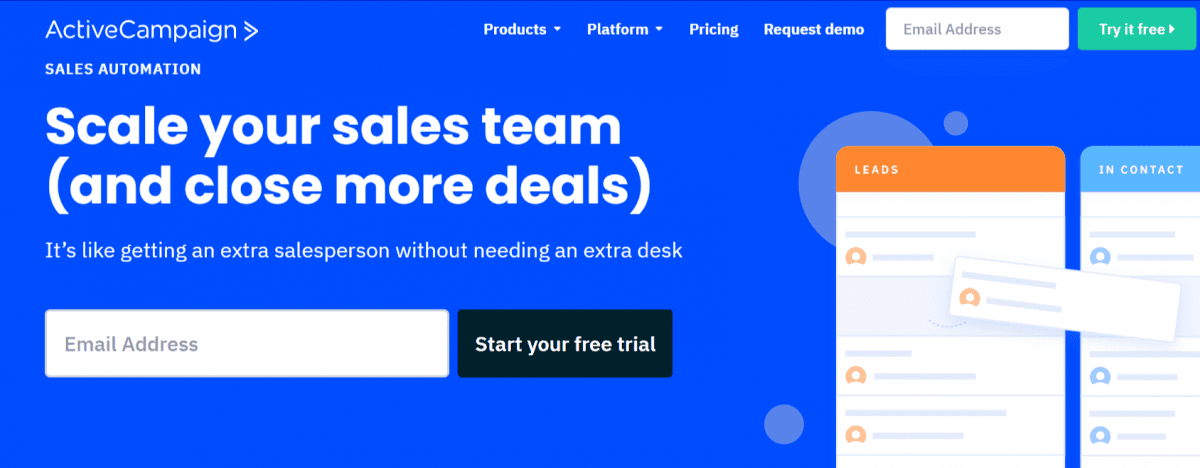This screenshot captures the homepage of ActiveCampaign, a comprehensive marketing automation platform. The web page prominently features options such as "Products," "Platform," "Pricing," and "Request Demo". A clear call-to-action buttons like "Start Your Free Trial" and "Try It Free" stand out, encouraging potential customers to experience the service without commitment. The page emphasizes sales automation, suggesting that users can "Scale Your Sales Team" and "Close More Deals," effectively adding an extra salesperson without the need for additional desk space. The site design incorporates a clean, professional aesthetic with a color palette of blue, white, orange, and green, enhancing the visual appeal and user experience. The email address field, currently empty, invites users to input their details to start a free trial or request a demo, further facilitating lead generation and customer acquisition.